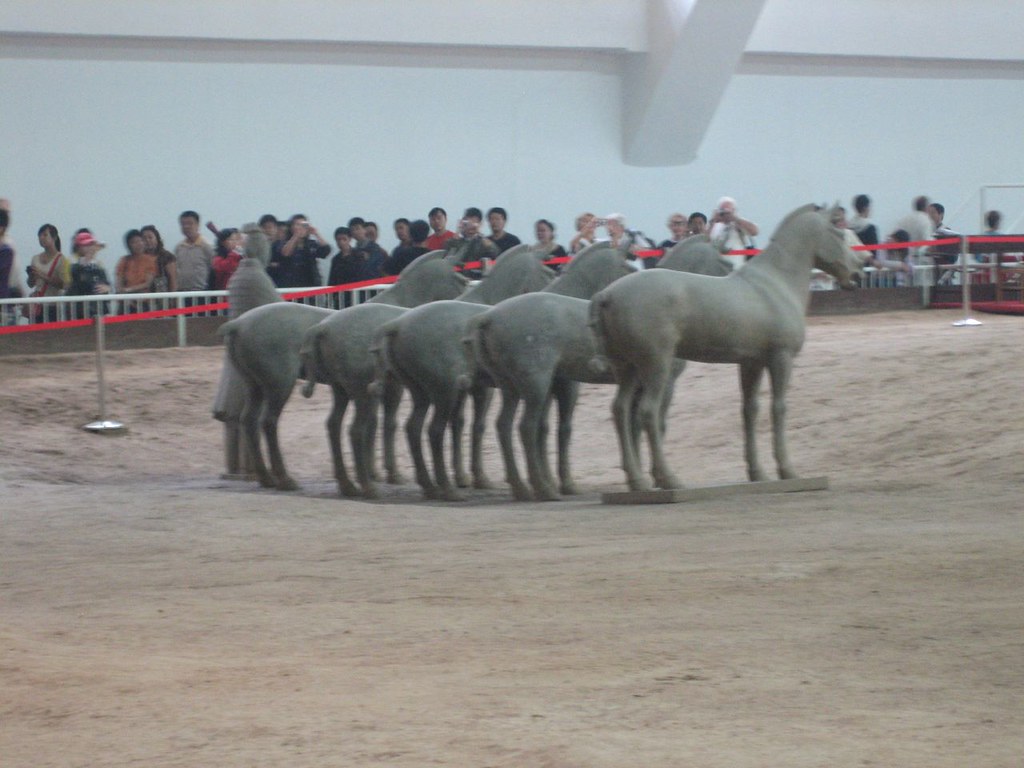The image depicts a group of five terracotta horse statues and an additional terracotta figure, resembling a Chinese dynasty figure, arranged in a sunken, dirt arena. They are encircled by a white fence with red ribbon barriers and metal posts, preventing the onlookers from getting too close. The crowd, consisting of people of various ages and ethnicities, some wearing hats, can be seen behind the fencing, taking photos with cameras and phones. The terrain where the statues stand appears to be slightly depressed, emphasizing the preserved nature of this historical display. The setting includes white walls with arches supporting the ceiling, suggesting an enclosed space likely dedicated to the exhibition of these ancient artifacts.